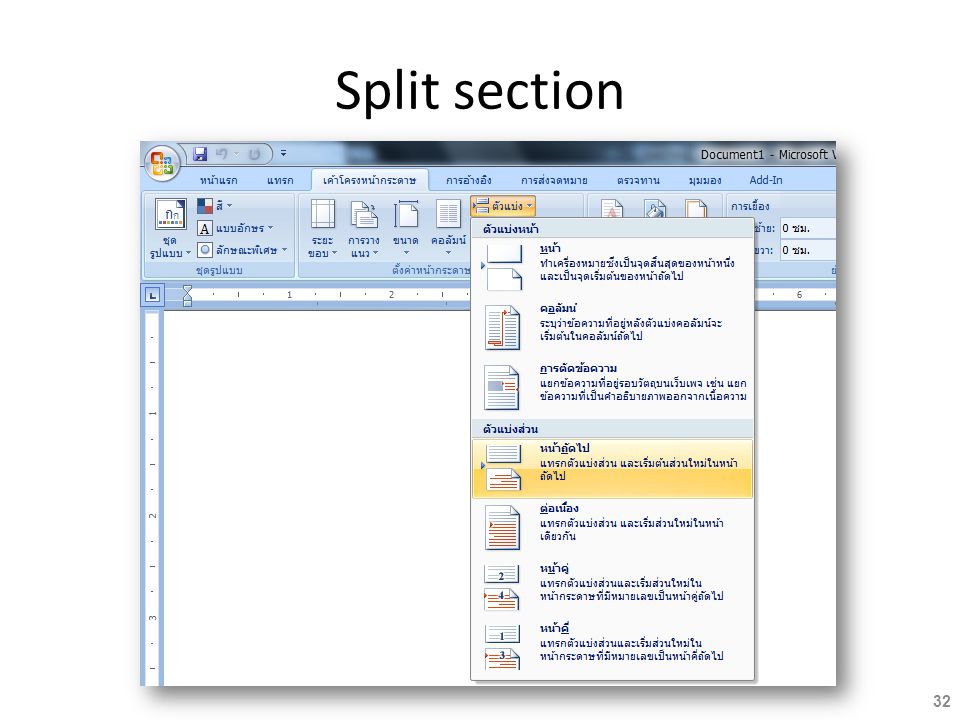The image depicts a screenshot of a Microsoft Word document interface with the "Split Section" feature highlighted in black font at the top. The interface language appears to be in Arabic. At the top of the screen, there's a blue section that includes the recognizable Microsoft Word logo on the left. The active tab on the ribbon is related to page orientation, displaying options for vertical and horizontal layout. A drop-down menu is visible, listing various selectable options. One specific item in the drop-down list is highlighted in orange, drawing attention to this selection within the interface. Although the language and specific details are unreadable, the visual context implies that the user is focusing on adjusting page layout settings.